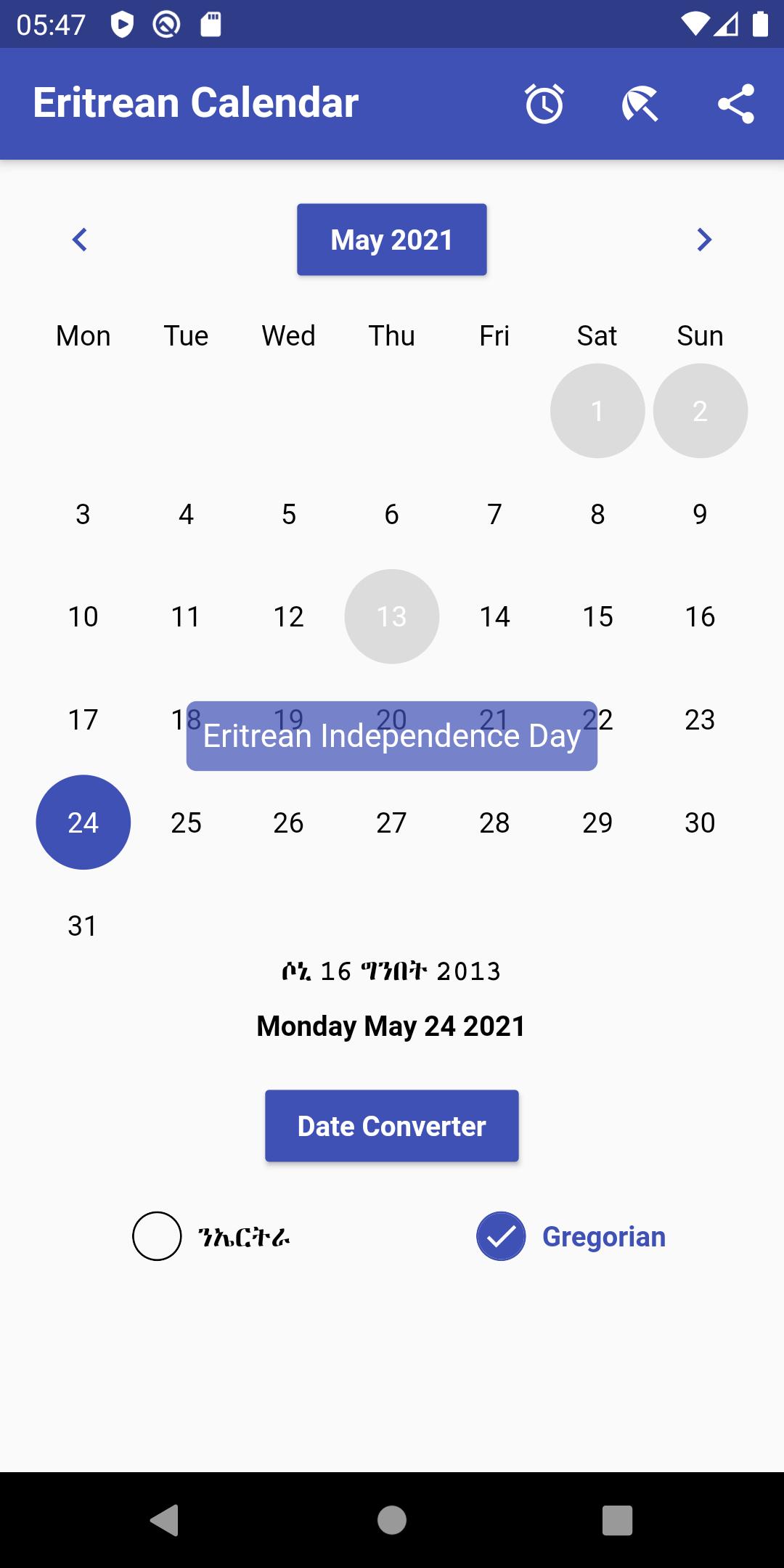This image is a screenshot of a mobile calendar application displayed in a vertical aspect ratio, indicative of a smartphone layout. The user interface is predominantly in a non-English language, although some elements are in English, illustrating a mixed-language setting. The screen features the typical mobile status bar at the top, showing icons for battery life, WiFi signal strength, volume, the current time, and active apps.

The calendar is set to May 2021 and prominently highlights Monday, May 24th, marking the Independence Day for a country named Etria. The application includes a button titled "Date Converter" and offers two selectable options: one labeled "Gregorian" and another in an undeciphered language and script.

At the bottom of the screen, the standard navigation buttons for back, home, and displaying all apps are visible, reflecting the typical layout found in many smartphone applications.